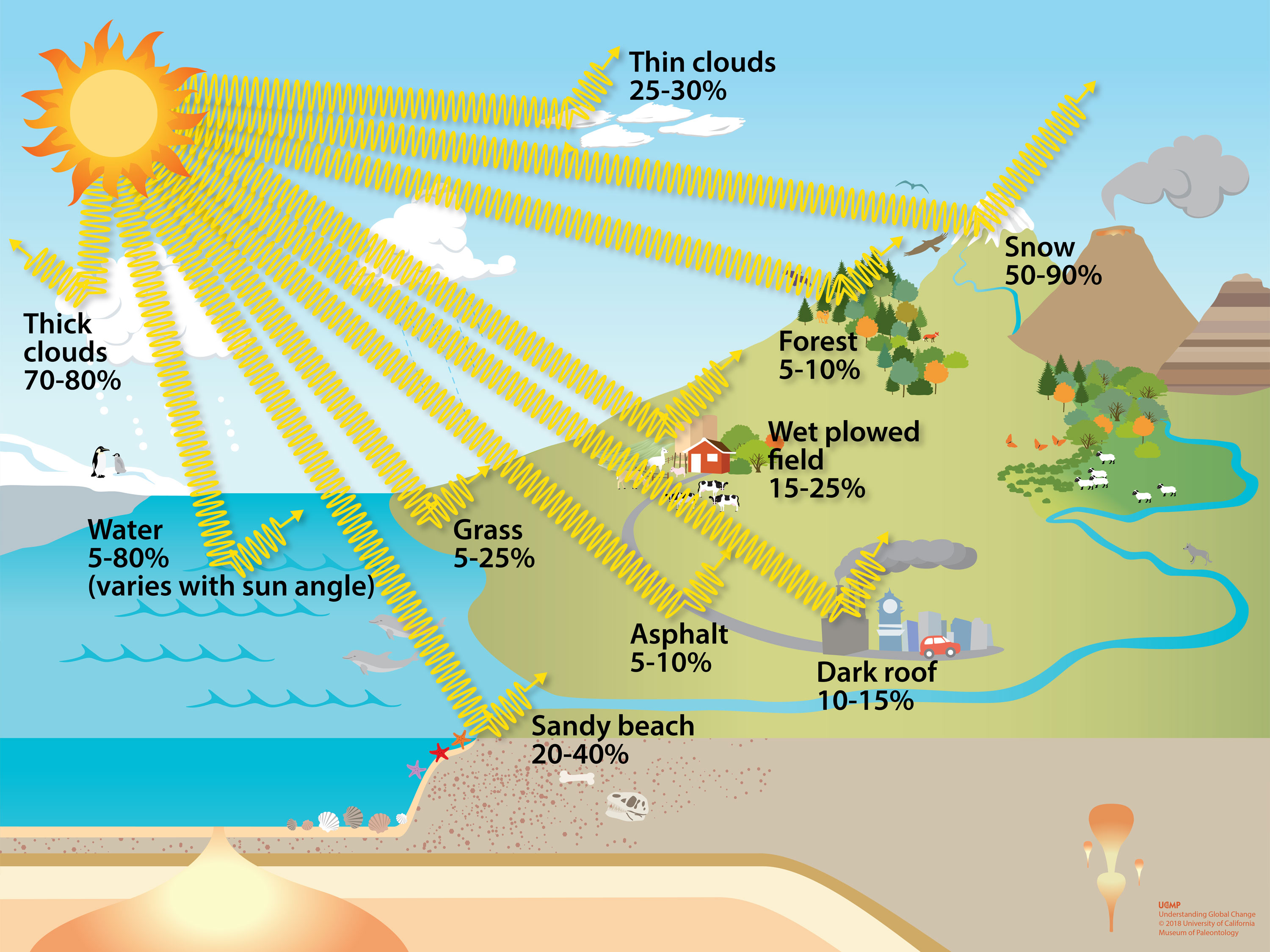This illustration is a detailed, computer-generated educational graphic, typically found in textbooks or notebooks, depicting how the sun’s radiation is distributed across various surfaces and objects during the daytime. The sun, located in the top left corner, extends its rays across a diverse landscape that includes a sky with clouds on both sides. The right side of the image showcases a vibrant, labeled scenery: grassy areas leading to forested regions, snow-capped mountains, sandy beaches, and a variety of urban and natural elements such as dark roofs, asphalt, and a wet plowed field. 

Each of these elements has specific labels indicating the percentage of the sun's rays they reflect or absorb. For instance, grass reflects 25%, sandy beaches reflect between 20-40%, dark roofs reflect 10-15%, asphalt reflects 5-10%, wet plowed fields reflect 15-25%, thick clouds reflect 70-80%, thin clouds have variable reflectance, and snow reflects 50-90%. An ocean and iceberg appear on the left, indicating water's reflective variation from 5-80% depending on the sun's angle. The graphic uses a spectrum of colors, including orange, yellow, blue, green, and brown, enhancing its educational value and clarity. This comprehensive visual representation elucidates the interaction between sunlight and different surfaces, illustrating how each element contributes to Earth's radiative balance and overall weather patterns.